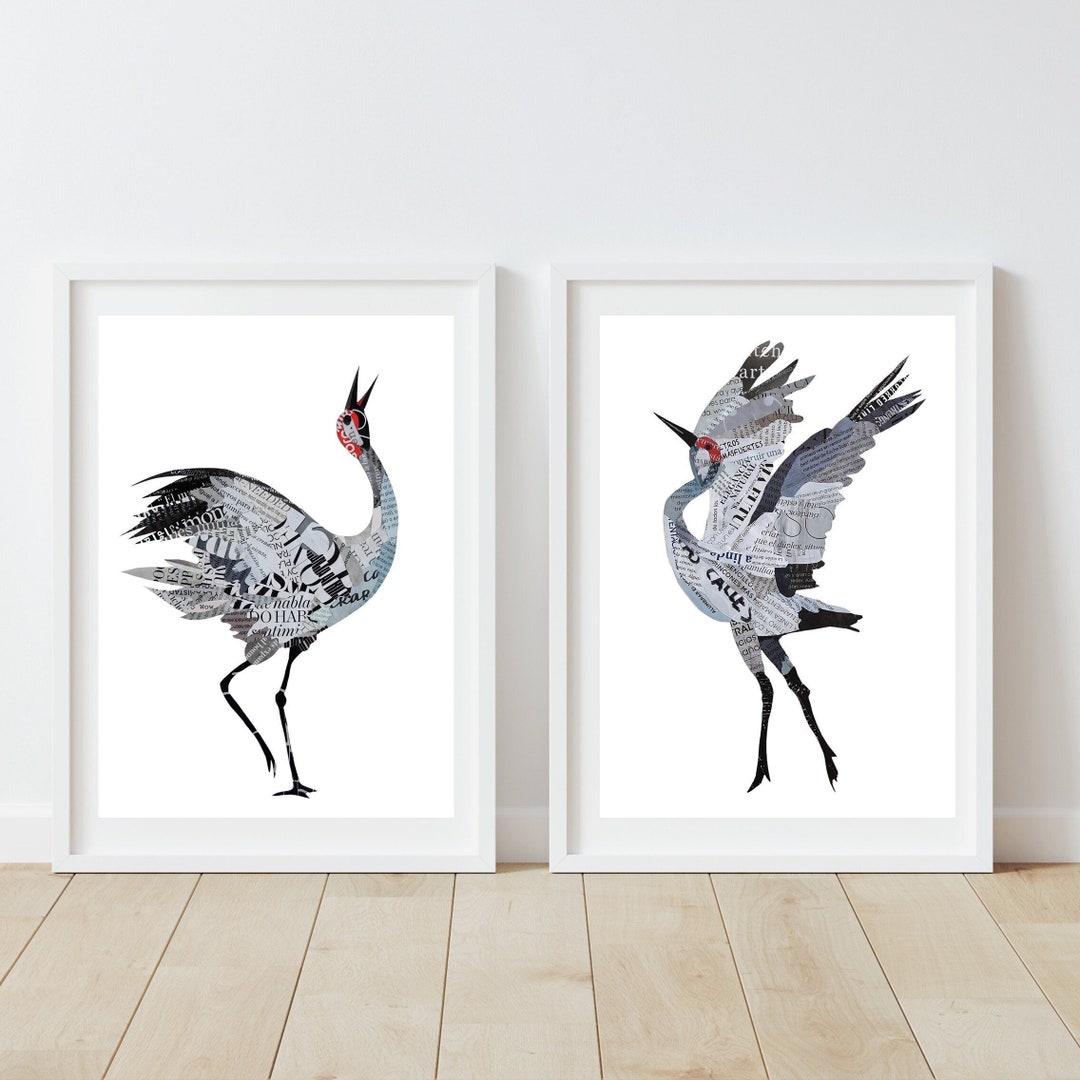In the photograph, two framed paintings rest on a light brown wooden floor, leaning against a light gray wall. The frames themselves are also a light gray color. The images within the frames depict intricately detailed birds crafted using paper cuttings, with a predominantly black and white palette accented by red areas around the birds' heads.

In the painting on the left, the bird's wings are closed, its head tilted upward with an open beak, suggesting a calling or singing posture. In the painting on the right, the bird's wings are spread wide open, its head also pointed upwards but angled towards the left, and its beak is closed. Both birds exhibit a graceful S-curve in their necks, adding a dynamic quality to their forms, as if they are in motion.

The left-side bird's leg is lifted, contributing to an impression of movement, while the right-side bird appears as though it has just leaped off the ground, with its toes pointed downward. The detailed feathers are depicted in shades of gray, with some darker streaks signaling the feather structures. The background of each painting is white, providing a stark contrast to the birds and highlighting the meticulous paper cutting technique used to create these lifelike representations of birds, likely whooping cranes.